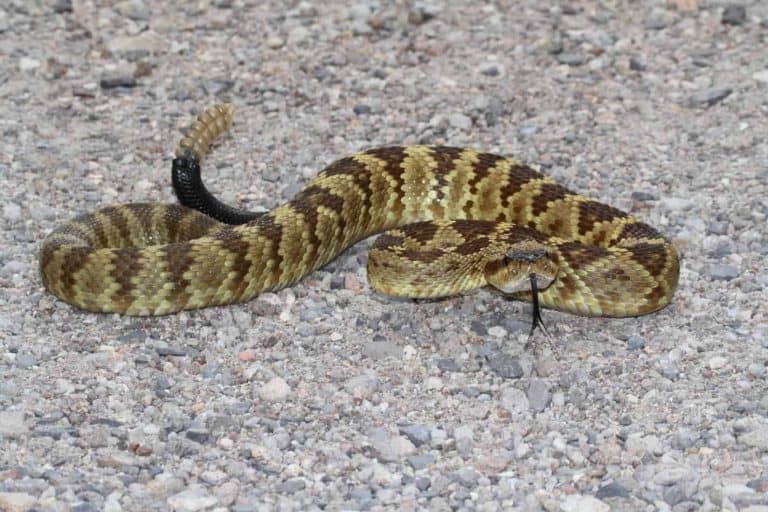In this close-up image, a snake is prominently featured in the center, lying on a gravel surface comprised of an array of differently sized and colored stones. The gravel is primarily dark gray, with some light gray, white, and brown pieces intermixed, creating a textured, multi-colored background. The snake itself displays an alternating pattern of dark brown and light brown bands, with hints of white along its body, adding to its striking appearance. The snake's head, small and positioned facing the viewer, contrasts with the thicker middle section of its body, which gradually narrows to a dark black tail tipped in beige. The reptile's scales are visibly detailed, enhancing its lifelike and slightly glossy, mucus-like light brown coloration. Coiled on the rocky surface, the snake's close-up portrayal captivates and directs the viewer's attention to its mesmerizing patterns and intricate textures.